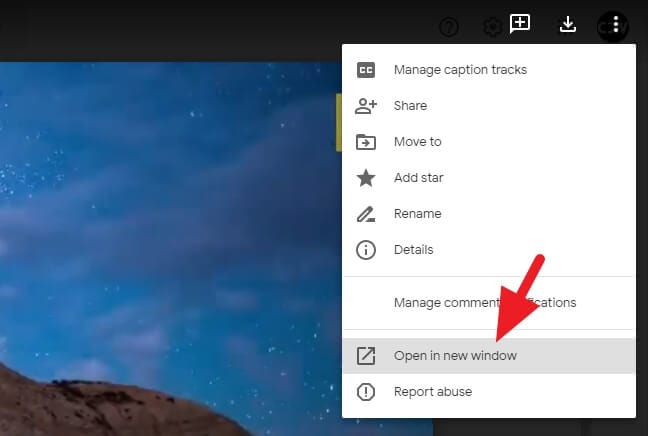In this image, the top section features a black toolbar containing a small white box with a plus sign, a down arrow next to a mint-colored line, and an icon with three vertical dots. The background is a clear blue sky, overlaying a large, brown, rocky hill, with several small white marks scattered across the sky. Below the toolbar, there's a white drop-down menu listing multiple options, each accompanied by its icon: "Manage Caption Tracks," "Share," "Move To," "Add Star," "Rename," and "Details." A thin gray line separates these options from another segment labeled "Manage Comments and Notifications," followed by another gray line. Further down, a gray box contains a smaller black box with a strikethrough line that reads "Open a New Window." This segment is highlighted by a large red arrow pointing at "Open a New Window." The drop-down menu also includes an option to "Report Abuse."